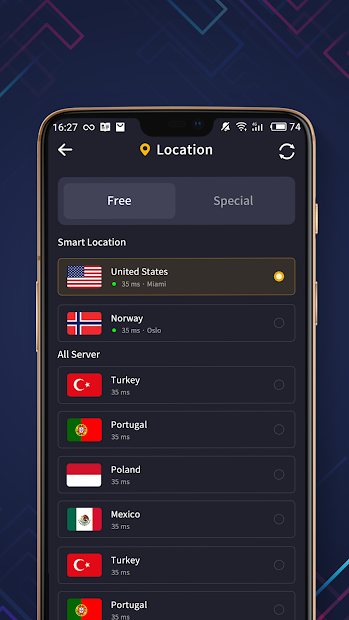The image depicts a phone screen set against a dark blue background adorned with pink and blue geometric lines creating abstract shapes on the left, right, and top edges. 

### Top of the Screen:
- **Time**: Displayed at 16:27 on the upper left.
- **Icons**: Three white icons next to the time.
- **Status Indicators**: On the upper right, there are icons for Wi-Fi, network connectivity, and a battery at 74% charge.

### Middle of the Screen:
- **Header**: The word "Location" is centered at the top.
- **Navigation Buttons**: To the left is a back arrow, and to the right is a refresh button.
- **Options**: Below the header are two tabs labeled "Free" and "Special."
- **List of Locations**:
  - **Primary Locations**: "Smart Location" is the category heading, with "United States" listed first and selected, indicated by a yellow dot within a dark brown rectangle. 
  - **Secondary Location**: Below the United States is "Norway," both with their respective flags to the left of the country names.

### Server List:
- **Title**: "All Servers" in white text.
- **Countries**: 
  - Turkey
  - Portugal
  - Poland
  - Mexico
  - Turkey (appears twice in the list)
  - Portugal (also appears twice, with the second instance at the bottom of the list)

Overall, the image comprehensively illustrates the structure and details of a location-selection interface on a smartphone, including the visual design elements and user interface components.